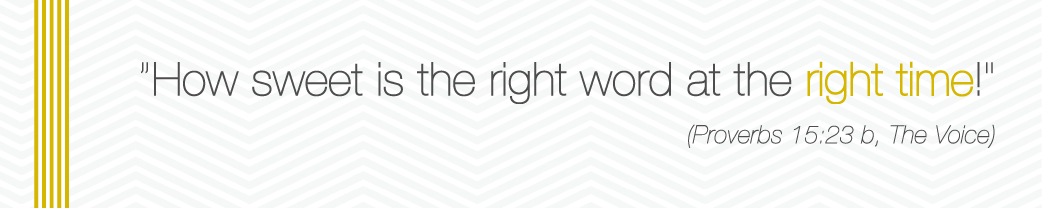The image is a wide, horizontal text-based graphic with a patterned background featuring light gray zigzagging lines on a white backdrop. On the left side, there are five vertical gold stripes. The central focus of the graphic is a quotation in a mix of light brown and gold text: "How sweet is the right word at the right time!" The words "right time" are highlighted in gold. Below the quote, in smaller light brown text and within parentheses, it reads "Proverbs 15:23b, the voice." The unusual aspect of the design is the thoughtful distribution of color and the sophisticated interplay of text and background patterns.